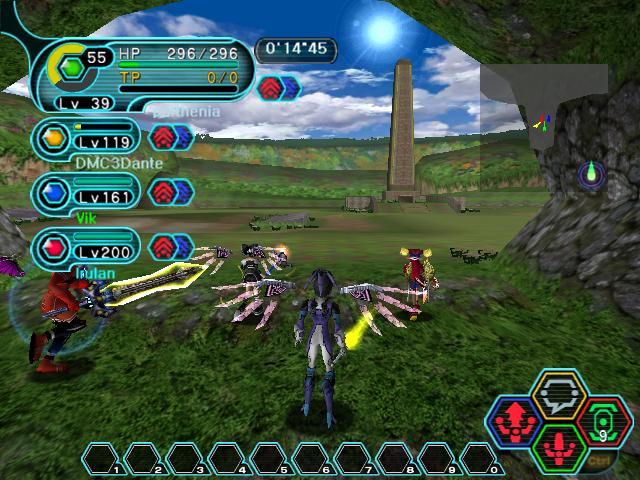In this detailed screenshot from an unidentified video game with somewhat blocky graphics, we find ourselves looking out from a dimly lit rock cave into a serene meadow. At the center of the view stands a tall stone monument, reminiscent of the Washington Monument, extending into the blue sky adorned with a glowing white sun and scattered white clouds. Beyond the monument, rolling green hills and valleys stretch into the distance.

In the foreground, closest to our perspective, is a prominently featured humanoid figure. This character, facing the viewer with their head slightly bowed, is equipped with large metal wings emerging from their back. They are dressed in a meticulous ensemble that includes a dark blue suit coat over a purple top, white pants, and striking purple boots with very high heels, which appear impractical for the grassy landscape. The character also sports a blue helmet and their leggings transition into blue boots. Hovering above each shoulder are their metallic grey wings. A faint yellow dust can be noticed near their right hand.

To the left of this primary figure, another character in red can be seen. This red figure wields a gold-edged sword that glows with a blue hue around their body, suggesting they might be in the midst of a battle. In the right-hand corner, another character, depicted in red and blue and holding weapons, adds to the scene's dynamic tension. Scattered in the foreground are three distinct objects in varying color combinations: orange with red, and purple with grey.

Overlaying the scene are numerous in-game informational elements. In the upper left corner, there are assorted numerical stats and indicators, such as player attributes like TP and HP, alongside levels for DMC Dante, VIK, and IRULAN. At the top, a time marker reads "0:14:45". The bottom right corner contains an array of icons, including four unidentified symbols, a chat box, an attack box, a sword icon, and a green square labeled with the number three. Additionally, colorful gems and directional arrows are also displayed.

Overall, this vibrant and detailed game screenshot immerses the viewer in a fantastical setting brimming with character interactions, battle indications, and a rich tapestry of on-screen information.